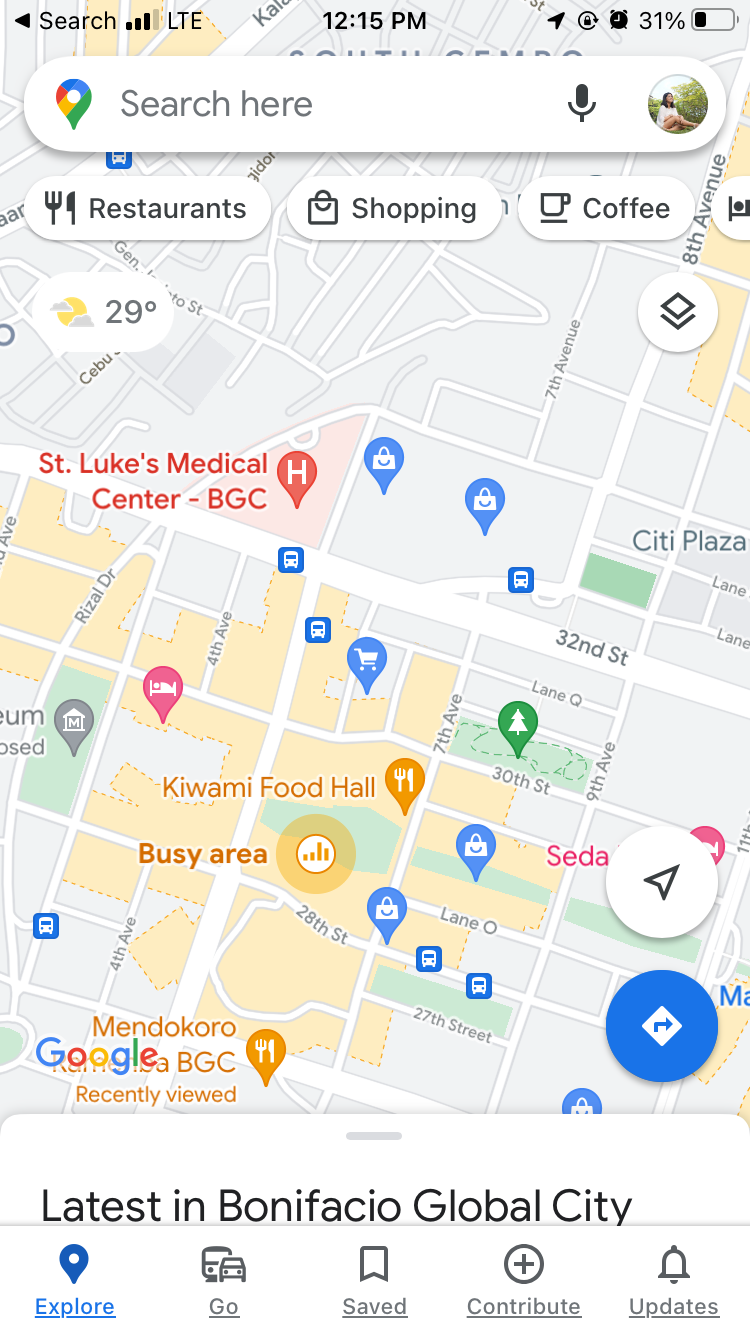This image is a screenshot of a cell phone displaying the Google Maps app. In the top left corner, there is a back arrow icon and a search bar with the words "Search here," accompanied by a microphone icon. The status bar at the top of the screen shows full cellular signal bars, an LTE indicator, the time "12:15 p.m.," an upload icon, an app icon, a clock icon, and the battery level at 31%.

Below the search bar are three tabs labeled "Restaurants," "Shopping," and "Coffee," respectively. These tabs are part of the map view, which shows an area under exploration. At the bottom of the screen, a banner reads "Latest in Bonifacio Global City," with an "Explore" button highlighted in blue. To the right of this button are options labeled "Go," "Saved," "Contribute," and "Updates."